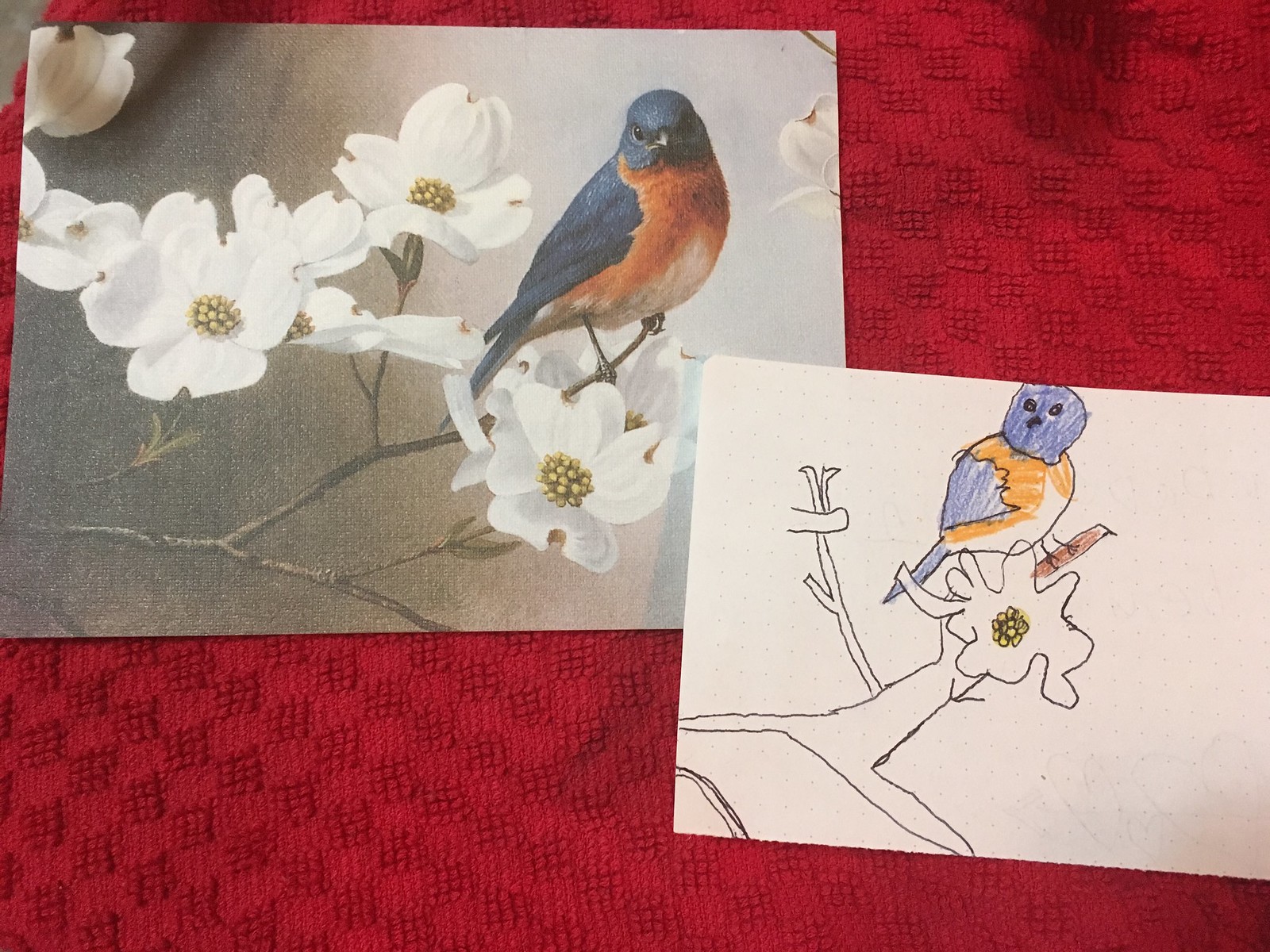In the image, there is a dynamically composed scene featuring a detailed painting and a child's drawing, both set against a textured red fabric background, which appears to be a dish towel. The painting is situated in the upper left corner and showcases a bird perched on a branch adorned with fully bloomed white flowers. Each flower has delicate, open petals and a light yellow center, likely representing pollen. The bird in the painting is meticulously depicted with a blue head and upper body, a burnt orange chest, and a small beak, closely resembling a robin.

Adjacent to the painting, in the lower right corner, is a child's drawing, partially overlapping the painting. This drawing is a simplified, yet earnest attempt to replicate the painting. It includes a sketch of the branch with one white flower and the bird. The bird in the drawing is colored with a blue head and wing, an orange belly, and is set against the textured red fabric background. The composition highlights the juxtaposition between the sophisticated detail of the painting and the charming simplicity of the child's drawing, both united by the vibrant red backdrop with its black and square patterns providing texture.